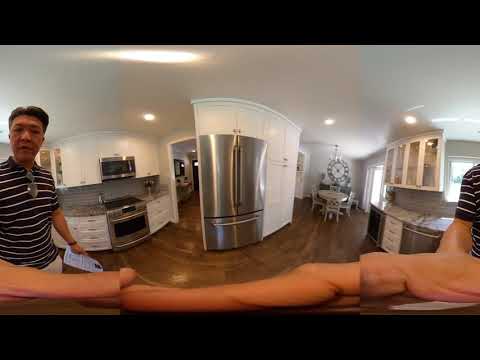This rectangular, panoramic photograph captures the interior of a contemporary kitchen, framed by black bands at the top and bottom edges. On the left side stands an Asian man with short dark hair, dressed in a black and white striped polo shirt with glasses tucked into the collar. He is holding a piece of paper. The kitchen backdrop features white cabinetry and stainless steel appliances, including a double-door refrigerator with a bottom freezer drawer at the center of the image, a stove with a built-in microwave above it to the left, and a dishwasher under a gray countertop on the right. The cabinets on the right wall have glass panel doors. The kitchen also includes a seating area on the far right with a white table and four chairs, set against a wall adorned with a large round clock. The space is finished with dark brown wood floors and a patio door, adding a touch of elegance to the modern design.